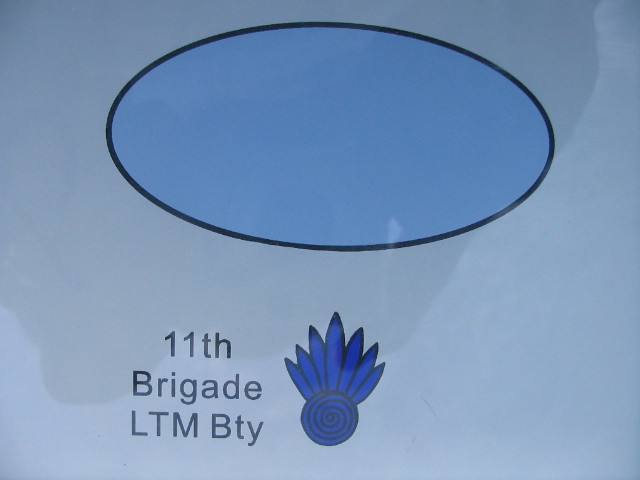The image portrays a glossy sign, likely taken outdoors, reflecting a faint silhouette of a person standing above it. The primary background is a light bluish-gray color, while a prominently featured oval sits centered at the top of the sign. This oval is slightly darker blue compared to the background, outlined with a black band. Below the oval, aligned slightly to the left, there is black text reading "11th Brigade LTM BTY" in clear, basic print.

Adjacent to the text is a distinct dark blue emblem. The emblem is a detailed drawing, showcasing a spiral-like swirl that loops several times before meeting at the center. Above the swirl, seven blue feathers are arrayed - three on each side and one larger feather in the center. The entire emblem is darker than the oval above and appears to be superimposed on the background. The background itself features a gray, watermark-like pattern that stretches diagonally downwards from the top, covering approximately two-thirds of the sign’s space.